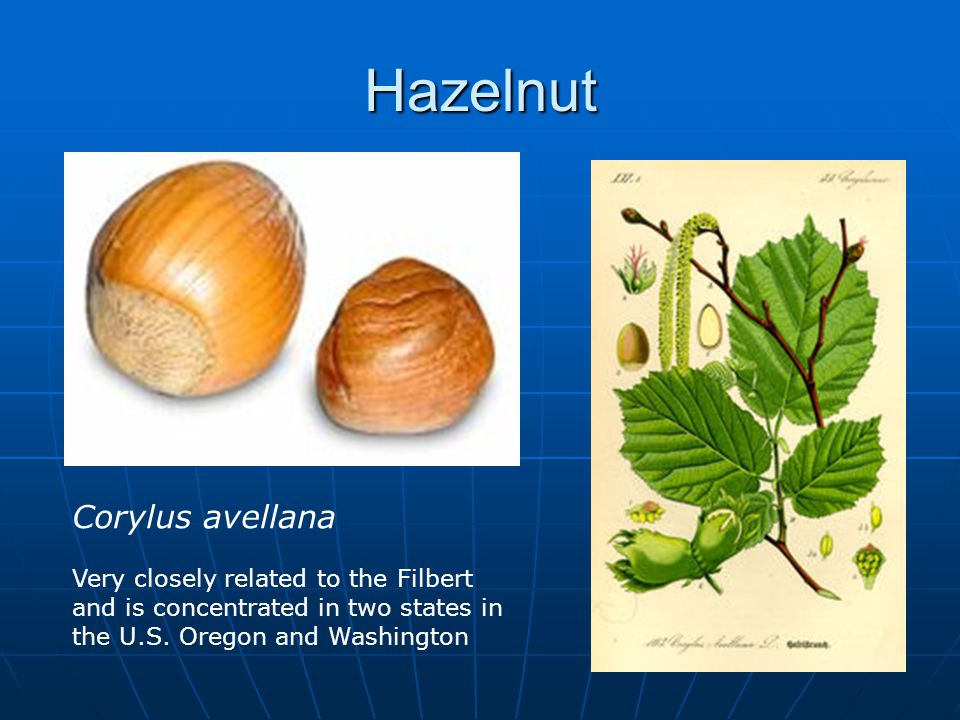This image features a detailed botanical presentation of the hazelnut (Corylus avellana) against a blue background. At the top, in white text, it reads "Hazelnut." On the left side, there's a section with a white background showcasing two brown, round hazelnuts. Beneath the hazelnuts, the Latin name "Corylus avellana" is displayed. It mentions that hazelnuts are closely related to filberts and are primarily found in Oregon and Washington. On the right side of the image, there's an illustration resembling a page from a botany book, depicting the hazelnut plant with green leaves, stems, and branches. This illustration includes a detailed look at the seeds and how they appear when sprouting. The bottom of the image contains additional text or a sentence, possibly in cursive, though it's not entirely legible. The overall composition resembles a slide from a PowerPoint presentation.